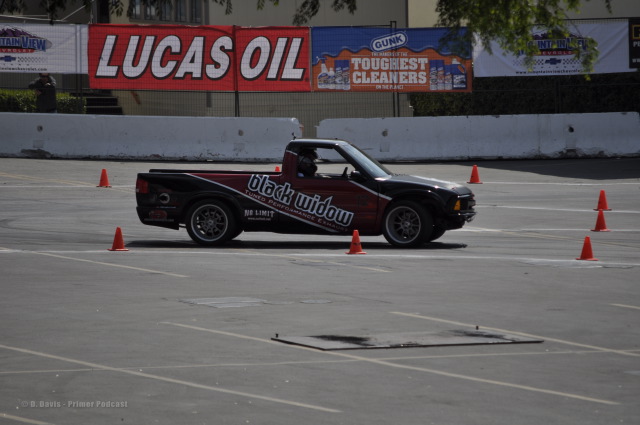The image depicts a well-worn asphalt surface, marked with faded white lines and multiple parking spaces, suggesting heavy usage over time. Positioned prominently is a large, black pickup truck adorned with a reddish stripe that spells out "Black Widow." The truck appears to be in a parking lot, surrounded by approximately seven traffic cones. Cement barricades, characterized by round rivets and minimal spacing between them, create a boundary around the area. Above these barricades is a fence lined with various advertisements, the most prominent being a red-and-white Lucas Oil sign with large, right-slanted white letters. Another notable ad promotes "Gunk, the Toughest Cleaner," featuring a small circular logo. Additional ads, though present, are less discernible, appearing primarily in green and white colors. The truck is the sole vehicle in the lot, and inside, a driver is faintly visible behind the wheel.